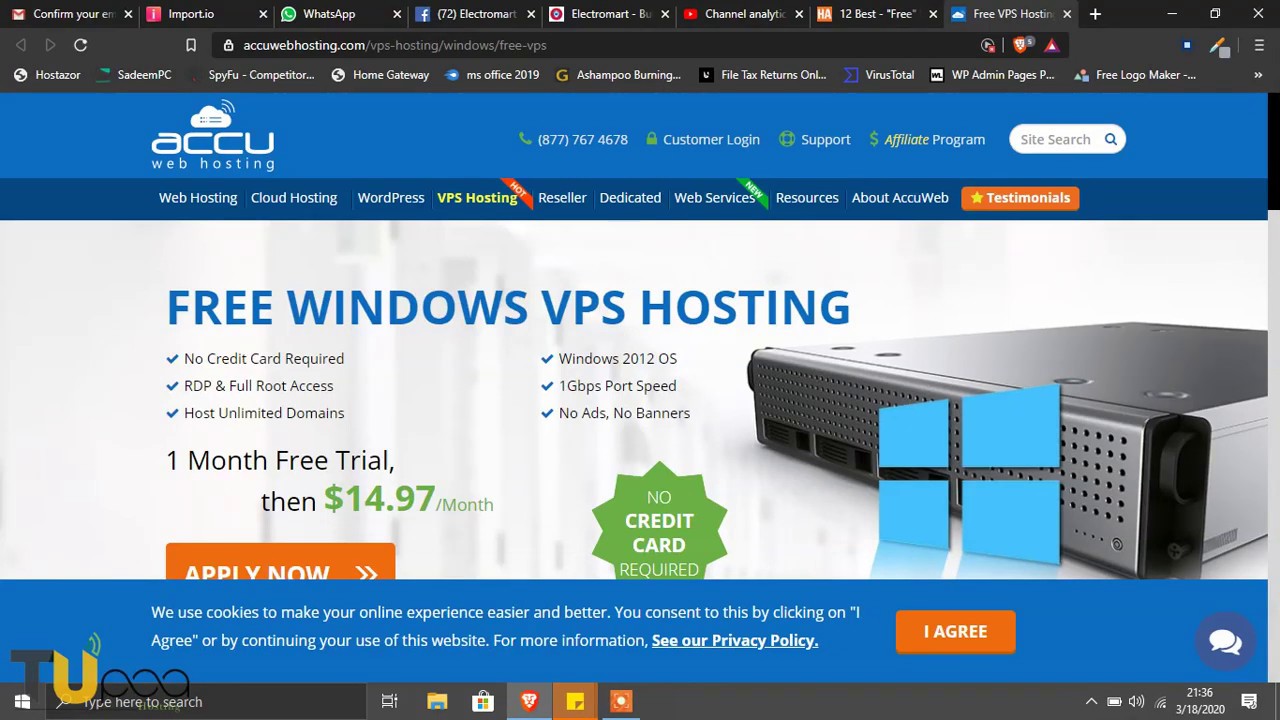The image depicts a web browser with a nighttime setting enabled, characterized by a black tint overlay. There are eight tabs open, with the focus on the far-right tab. At the top of the browser, a light blue border is visible, displaying the text "ACCU," accompanied by a phone number, customer login, and support options. Adjacent to this, there is a search bar.

Below the light blue border, a darker blue navigation bar lists various options including web hosting, cloud hosting, WordPress, VPS hosting, reseller, dedicated, web services, resources, and information about AccuWeb. Additionally, there is an orange box labeled "testimonials."

The main section of the webpage features a white background with bold blue capital letters announcing "FREE WINDOWS VPS HOSTING." An image of a metallic box with the Windows logo is displayed prominently. Against a green background, the text states "No credit check, no credit card required." Accompanying this message is an orange button with "APPLY NOW" inscribed in white capital letters.